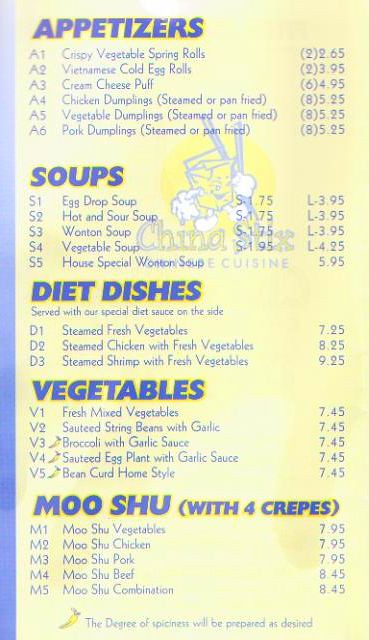This image showcases a detailed menu set against a vibrant yellow background with blue accents. The menu is divided into several sections with blue font conveying the dish names and descriptions.

At the top is the "Appetizers" section, which includes:
- **A1 Crispy Vegetable Spring Rolls** (2) - $2.65
- **A2 Vietnamese Cold Egg Rolls** (2) - $3.95
- **A3 Cream Cheese Puffs** (6) - $4.95
- **A4 Chicken Dumplings** (Steamed or Pan-Fried, 8) - $5.25
- **A5 Vegetable Dumplings** (Steamed or Pan-Fried, 8) - $5.25
- **A6 Pork Dumplings** (Steamed or Pan-Fried, 8) - $5.25

Following this section is "Soups," offering:
- **S1 Egg Drop Soup** (Small $1.75, Large $3.95)
- **S2 Hot and Sour Soup** (Small $1.75, Large $3.95)
- **S3 Wonton Soup** (Small $1.75, Large $3.95)
- **S4 Vegetable Soup** (Small $1.95, Large $4.25)
- **S5 House Special Wonton Soup** - $5.95

Next, the "Diet Dishes" section highlights health-conscious options, served with a special diet sauce on the side:
- **D1 Steamed Fresh Vegetables** - $7.75
- **D2 Steamed Chicken with Fresh Vegetables** - $8.25
- **D3 Steamed Shrimp with Fresh Vegetables** - $9.25

The "Vegetables" section lists:
- **V1 Fresh Mixed Vegetables** - $7.45 
- **V2 Sautéed String Beans with Garlic** - $7.45 
- **V3 Broccoli with Garlic Sauce** (Pepper symbol indicating spiciness level can be adjusted) - $7.45 
- **V4 Sautéed Eggplant with Garlic Sauce** (Pepper symbol) - $7.45 
- **V5 Bean Curd Home Style** (Pepper symbol) - $7.45

Finally, the "Mushu" section, which includes four crepes with each dish, offers:
- **M1 Mushu Vegetables** - $7.95
- **M2 Mushu Chicken** - $7.95
- **M3 Mushu Pork** - $7.95
- **M4 Mushu Beef** - $8.45
- **M5 Mushu Combination** - $8.45

At the bottom of the menu, a legend indicates that dishes marked with a pepper symbol can have their degree of spiciness adjusted according to preference.